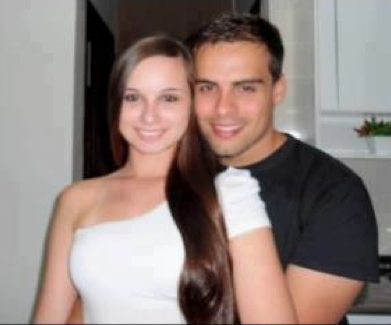In the image, a man and a woman stand close together, facing forward, with the man's head gently resting against the woman's face. The man, positioned on the right side, is dressed in a black shirt and has dark brown hair. The woman, with long brown hair flowing below her chest, partially covers her left shoulder with her hair, leaving it bare, while her right shoulder is covered by her dress. The woman's hair creates a visual illusion, making it appear as though the man's arm, which disappears behind her, is actually an amputated arm with a bandage at the end. This optical illusion is due to the way her hair separates the view between her chest and shoulder, giving the impression that his arm bends and points towards his chin.